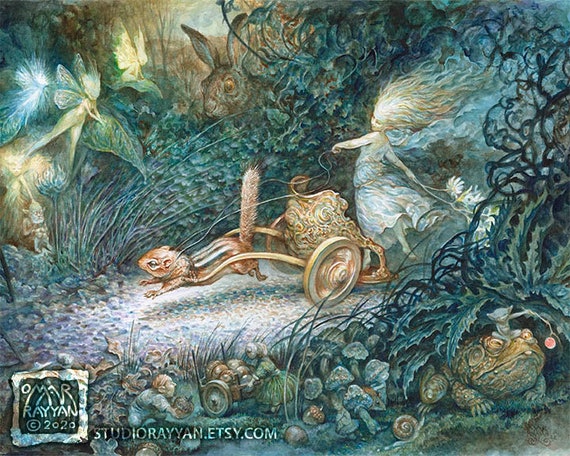This detailed fantasy scene painting reveals a vibrant forest area filled with whimsical elements. Dominating the composition is a golden chariot driven by a brown squirrel, depicted from a side view. A young girl, dressed in a flowing blue gown with her hair whipping back from the motion, stands on the chariot holding the reins and white flowers, which might also act as a whip. Surrounding the chariot is lush greenery with various fantastical creatures: a rabbit and a frog are hidden among the plants, along with small fairies flying in the air. Additionally, there are miniature people or dwarfs engaged in various activities, such as pulling wooden carts laden with fruits. A vine arch, tightly wound with leaves, sits prominently on the right side of the scene, providing an entryway to this enchanting world. At the bottom left corner of the image, a logo resembling a vintage photo frame reads "Omar Ryan, 2020," and the artist’s website, "studiorayon.etsy.com," can be seen. This multifaceted artwork combines fairytale charm with intricate natural details, inviting the viewer into a magical narrative.